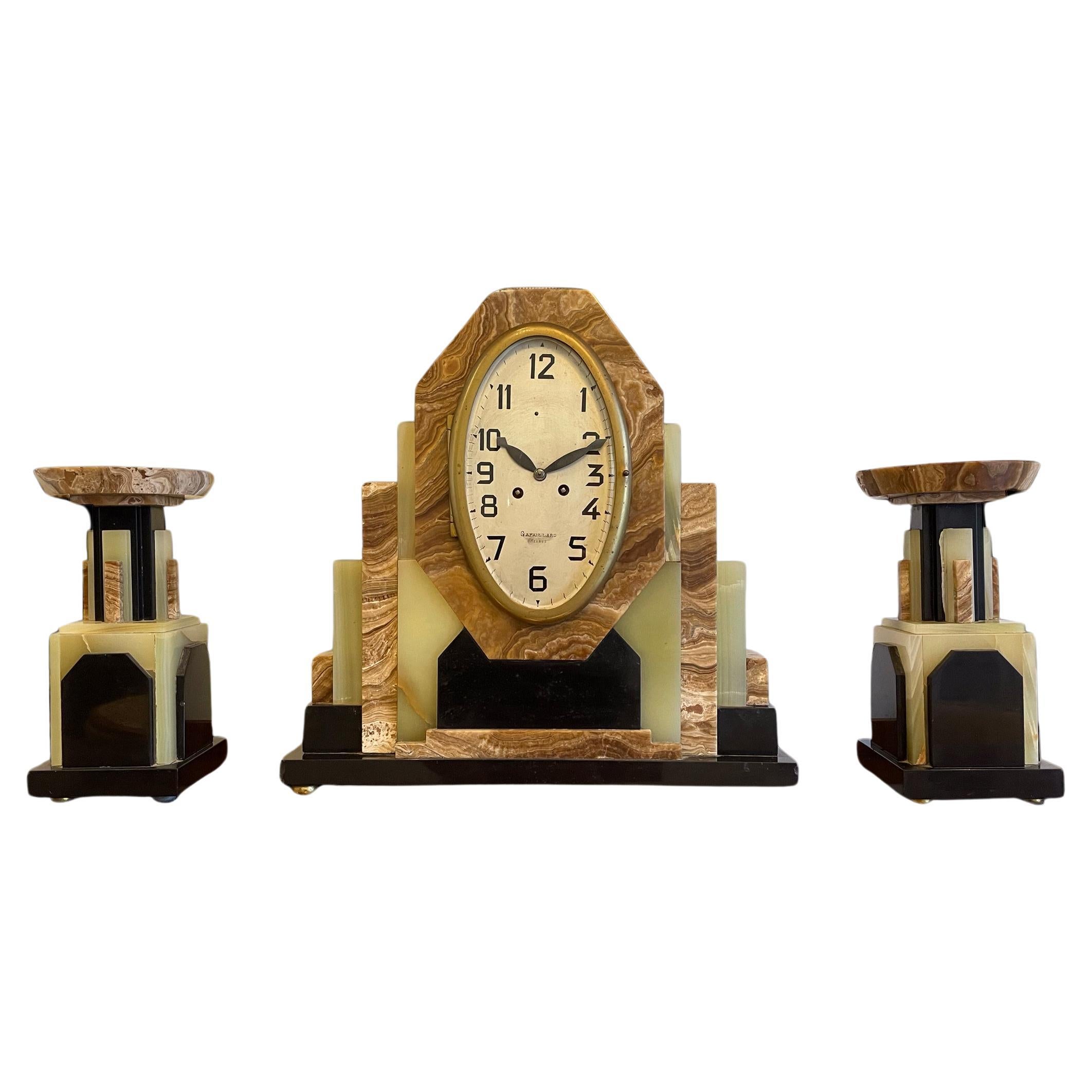In the center of this detailed photograph stands a solid, antique clock, intricately built into an exquisitely crafted series of marble plinths. The marble structure exhibits multiple levels of elevation, with the larger base plinth supporting an octagonal oval plinth that holds the actual clock face. The clock, which is showing the time as 10:10, features a minimalistic design with a narrow oval face, displaying both minute and hour hands, but no second hand, and all the numbers are clearly visible. Flanking the clock on both sides are two identical bookend-like objects that resemble trophies. These objects have a rectangular prism base made of marble, with darker panels on the sides, and supporting wooden cups atop. The clock and its accompanying pieces share a consistent color palette of cream, brown, black, and a quartz-like texture, setting a sophisticated visual symmetry against the stark white background.